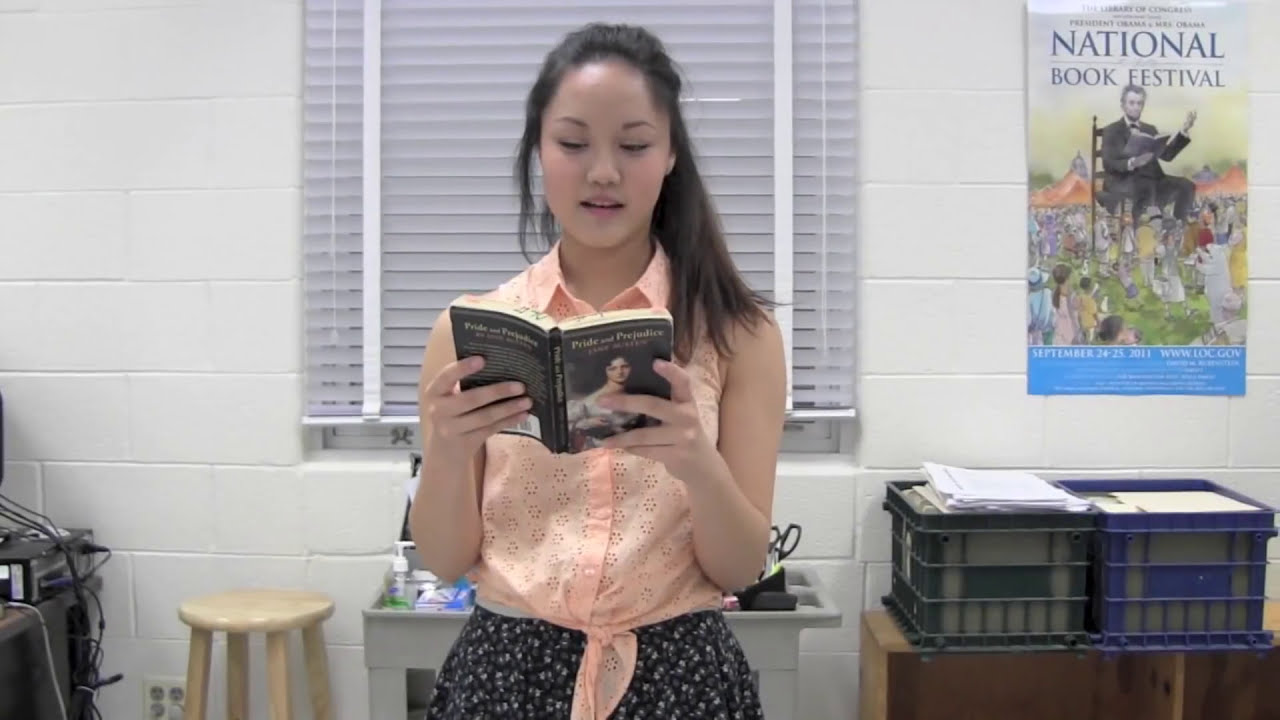In this image, a woman is standing in a brightly lit room, likely a classroom, in front of a white cinder block wall with a fully closed white blind on a window. She has long black hair tied back in a ponytail and a lighter skin complexion. She is holding a paperback book titled "Pride and Prejudice" with both hands, gazing down at it as she reads. She is dressed in a pink, sleeveless, button-up blouse and a black skirt adorned with small white designs. To her right, a colorful poster featuring the text "National Book Festival" in blue letters hangs on the wall, depicting a cartoon image of Abraham Lincoln sitting in a large chair, reading a book aloud to a group of children. Also visible in the background is a grey cart holding various office supplies such as sanitizer and scissors. The camera is positioned approximately four feet from her, capturing her from the waist up.